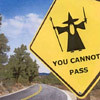This extremely diminutive image, measuring approximately one inch by one inch, showcases an outdoor scene. Due to its minimal size, it is difficult to determine if it is a photograph or a graphic. In the upper left corner, the scene unfolds with a blue sky adorned with scattered clouds. Transitioning to the lower left section, lush trees come into view, contributing to the outdoor ambiance. Dominating the central lower part of the image, a road extends forward, guiding the viewer's eye to the focal point. Occupying nearly half of the image, a cube-shaped sign, precariously set on its axis, captures attention. This yellow sign features a striking black silhouette of Gandalf from "The Lord of the Rings," accompanied by the iconic phrase "You Cannot Pass" in bold black font beneath the silhouette.